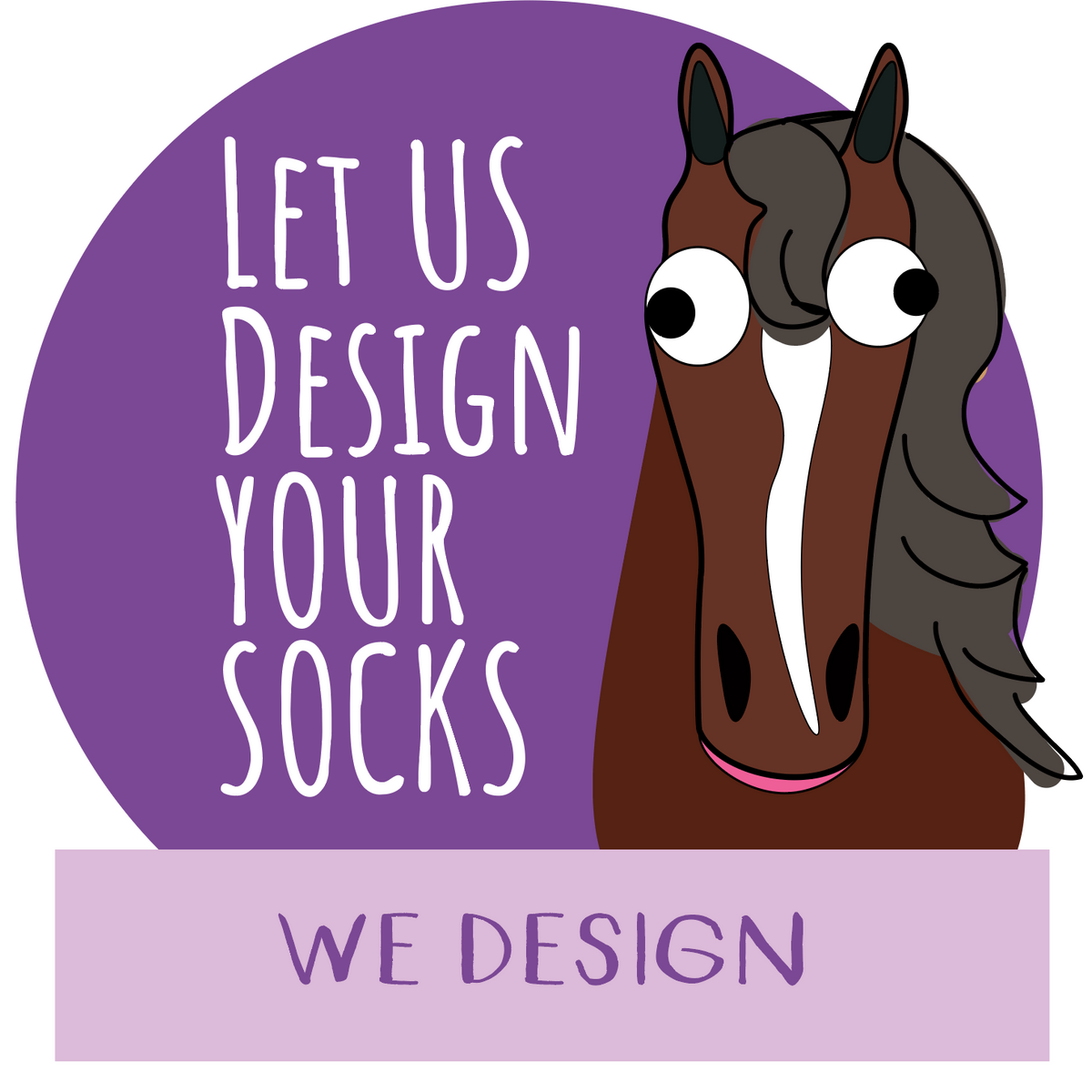The advertisement features a striking design with a large, dark purple circle as the central element. Within this circle, positioned towards the right, is a cartoon drawing of a horse. The horse, predominantly brown with a distinctive white stripe running down the center of its face, has a black mane, black inner ears, black eyes, and a pink crescent-shaped mouth that appears wide open, giving it a quirky, googly-eyed expression. Its eyes are colored blue-grey, adding to its unique appearance. The text "Let us design your socks" is prominently displayed in white within the purple circle. Below the circle, there's a light purple rectangle banner featuring the word "redesign" in purple text. This combination of geometric shapes, text, and the distinctly drawn horse makes for an eye-catching and whimsical graphic design.